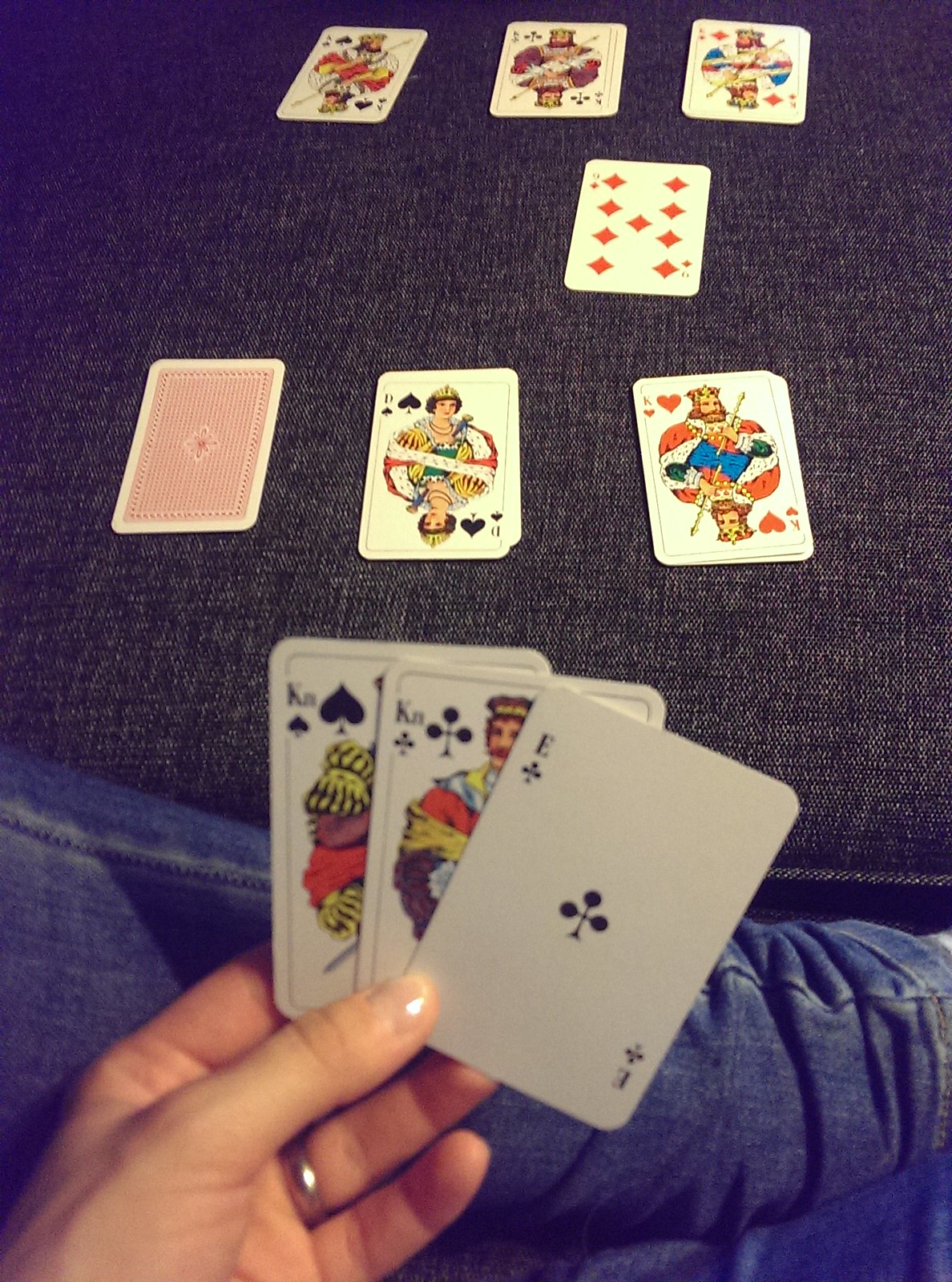A person is seated, balancing their left leg across their right knee. They are holding three playing cards in their left hand, showcasing a silver ring on their ring finger. The cards they hold include an "E" card with a club symbol in the center, and two kings, each adorned in regal attire featuring purple, gold, and red. 

In front of them are seven piles of cards. The arrangement consists of three cards face-up in the back row, one in the middle, two face-up on the front right side, and one face-down on the far left. The face-up cards reveal a queen wearing a crown, another king, a diamond card, two more kings, and another queen. The face-down card displays its red back.

The setting includes a blueish jean-like cushion, which complements the person’s blue skinny jeans.